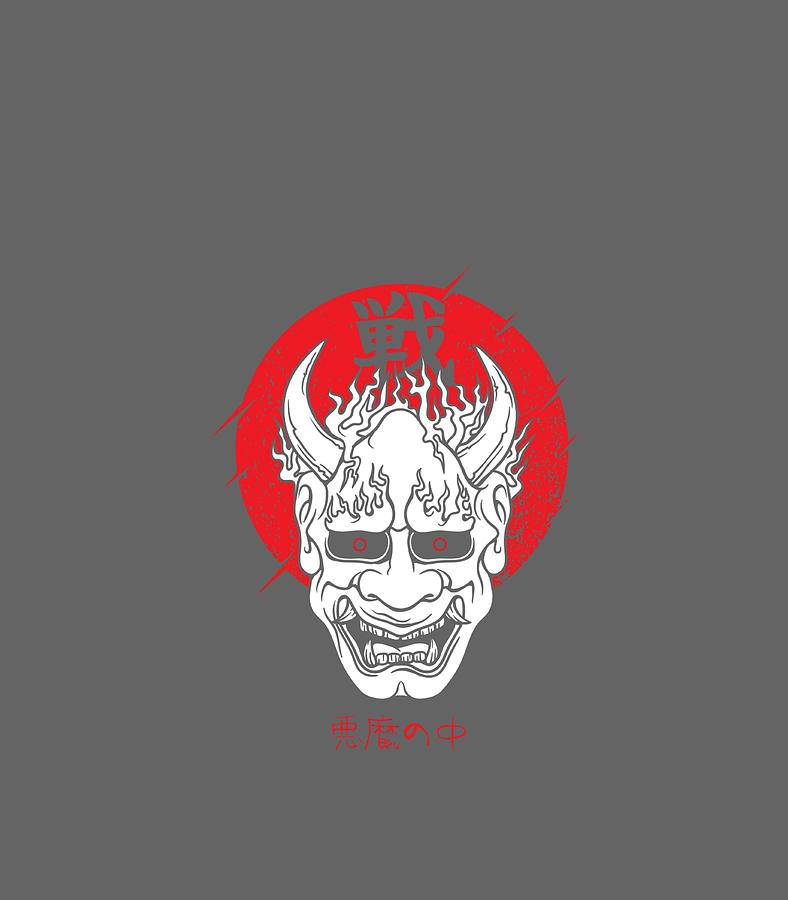The image is a detailed Japanese-style woodblock print featuring a demon head centered against a slate gray background. The demon, primarily white with gray accents, has an imposing visage with wild, flame-like hair, two prominent horns on either side of his forehead, and large, pointed ears. His eyes are gray with bright red pupils that appear hollow. His mouth, open in a menacing grin, displays sharp canine-like teeth on both the upper and lower jaws, resembling a vampire's fangs. A distinctive cleft marks his chin.

The demon is encircled by a vibrant red circle with jagged edges, adding to the sense of intensity. Surrounding the red circle are small, intricate lines extending outward. Above the demon's head, within the red circle, are gray Japanese Kanji characters. More red Japanese characters appear beneath the demon's head, with some of the text decipherable as “no naka,” which potentially refers to "the center." The overall visual evokes a sense of eerie folklore, further emphasized by the ancient and mystical symbolism embedded within the illustration.